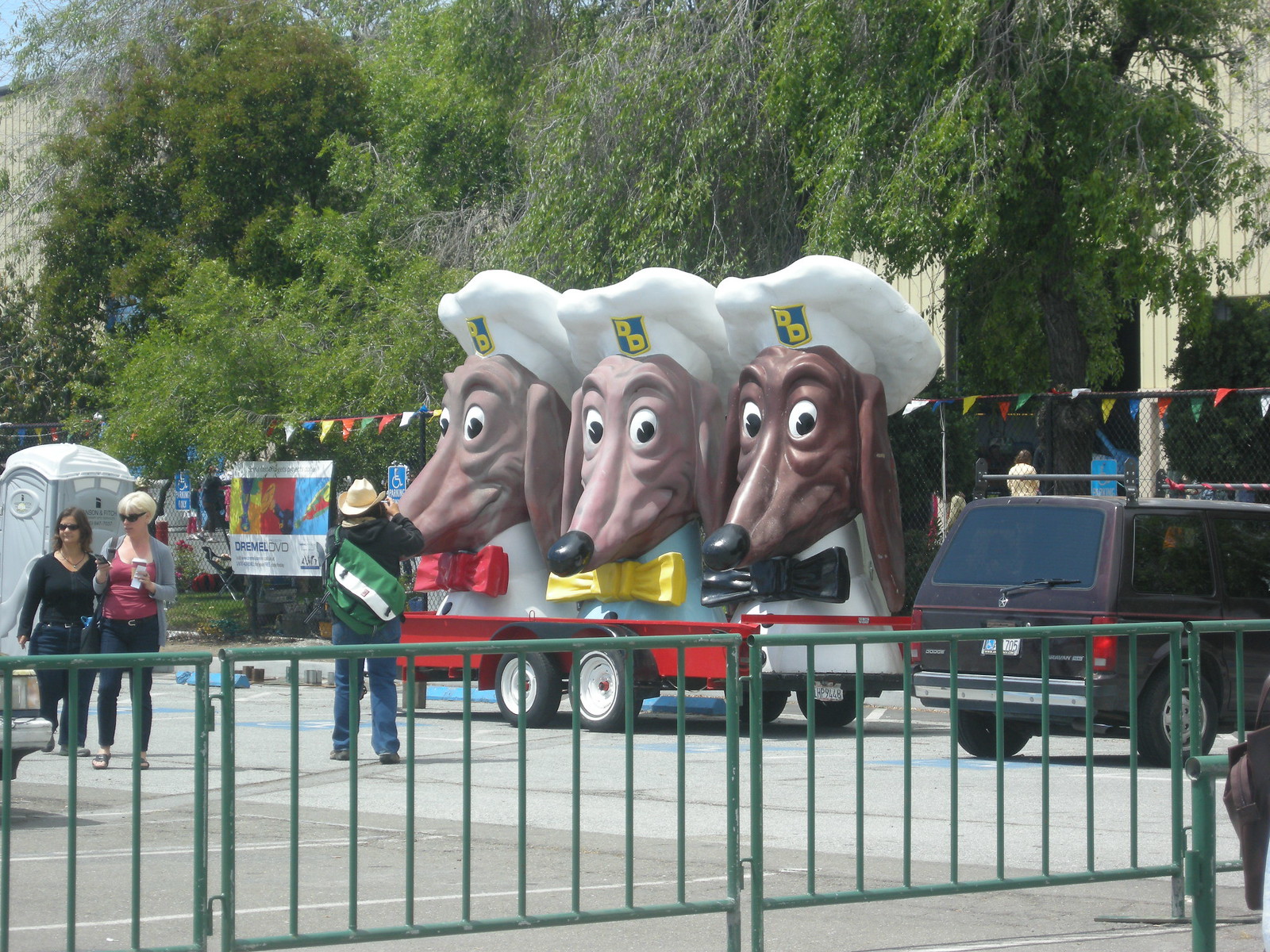This outdoor color photo showcases a whimsical parade or carnival scene featuring a trailer adorned with three large dachshund heads. Each of the dachshunds sports a puzzled expression, with brown faces, varying shades of noses, and prominent white eyes featuring black pupils. They are dressed in white chef outfits complemented by colorful bow ties—red, yellow, and black respectively—and top their look with large white chef hats marked by a green square emblazoned with "DD" in yellow lettering.

The backdrop presents a tan-colored building against a medium-toned blue sky, and a densely packed line of medium green trees beneath it. There is an SUV near the trailer, emphasizing the bustling environment. In the foreground, the scene is enclosed by a green metal fence, past which a man, clad in jeans, a black shirt, and a green-and-white backpack, is seen photographing the quirky display. Two women, one in jeans and a black shirt and the other in jeans, a red shirt, and a gray sweater, walk in the opposite direction. Additionally, a gray port-a-potty is visible in the upper left corner, adding to the lively outdoor setting.